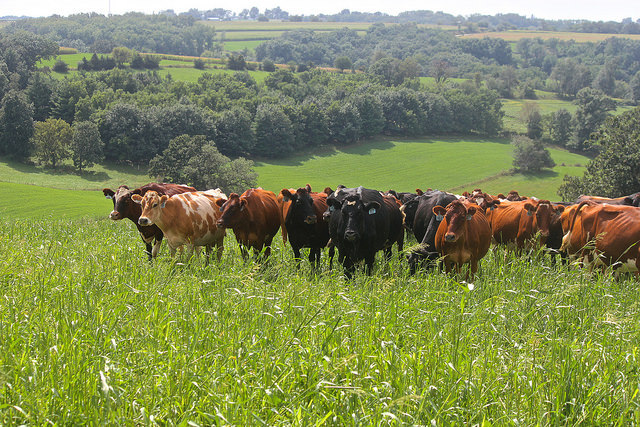The photograph captures a picturesque scene on a hillside meadow filled with a herd of approximately two dozen to forty cows. The cows, varying in color from dark brown and black to spotted white and brown, are some facing the camera while others graze in the tall, foot-high green grass. Visible tags dangle from each cow's ears. The meadow stretches out with more cows dotting the descending hillside. The background features rolling hills adorned with fields of grass and dense clusters of tall trees, their leaves vibrant green under a bright yet cloudy, slightly overexposed sky. There's a serene, foggy distant horizon adding to the tranquil rural landscape.